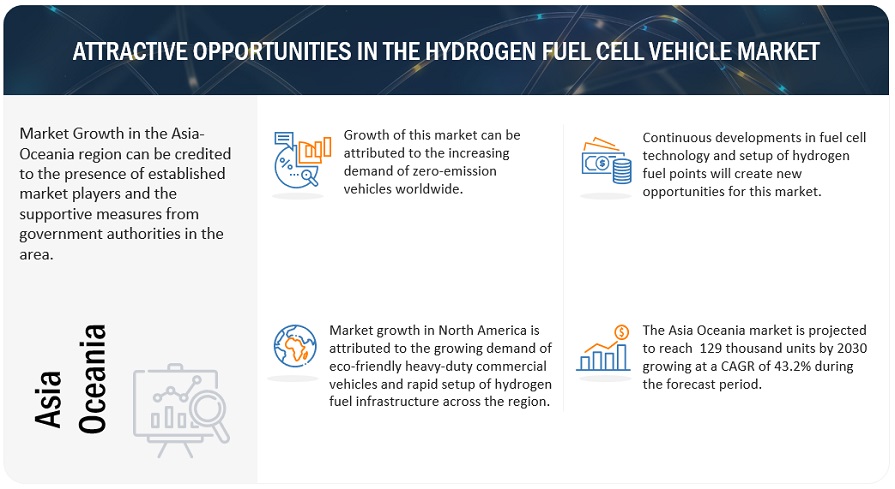The image appears to be a stylized digital art or poster board resembling a pamphlet, designed to highlight attractive opportunities in the automotive fuel cell market. The top banner, featuring a blue background with light or signal motifs, prominently displays the title "Attractive Opportunities in the Automotive Fuel Cell Market." 

The layout is divided into three main sections:
1. **Left Section:**
   - **Header:** Vertical text stating "Asia-Oceania" accompanied by a clip art of a board with graphs.
   - **Content:** Discusses the market growth in the Asia-Oceania region, attributing it to established market players and supportive governmental measures. The region is projected to reach 129,000 units by 2030, growing at a CAGR of 43.2% during the forecast period.

2. **Center Section:**
   - Details the growth of the fuel cell market, primarily driven by the increasing demand for zero-emission vehicles worldwide.

3. **Right Section:**
   - Elaborates on the market growth in North America, citing the growing demand for eco-friendly heavy-duty commercial vehicles and the rapid establishment of hydrogen fuel infrastructure.
   - Further mentions that continuous advancements in fuel cell technology and the setup of hydrogen fuel points are expected to create new opportunities in the market.

Each section is visually enhanced with relevant clip art to attract attention and emphasize key points.